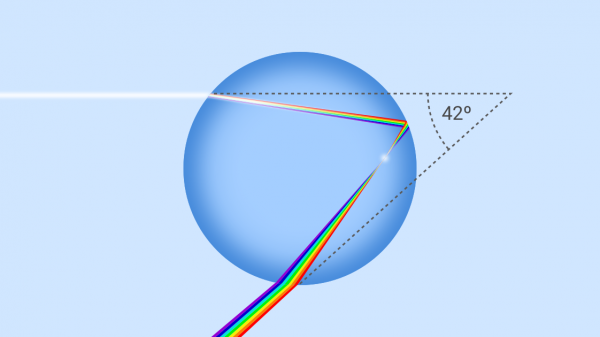The image shows a scientific diagram set against a pale blue background. At the center, there is a darker blue sphere. On the top left of the sphere, a beam of light enters and transforms into a rainbow pattern as it passes through the sphere. This rainbow light exits the sphere on the bottom right side, slightly bending as it does so. The diagram includes a dashed gray line indicating the angle of refraction, measured at 42 degrees, with each leg of the angle touching the sphere where the light changes direction.